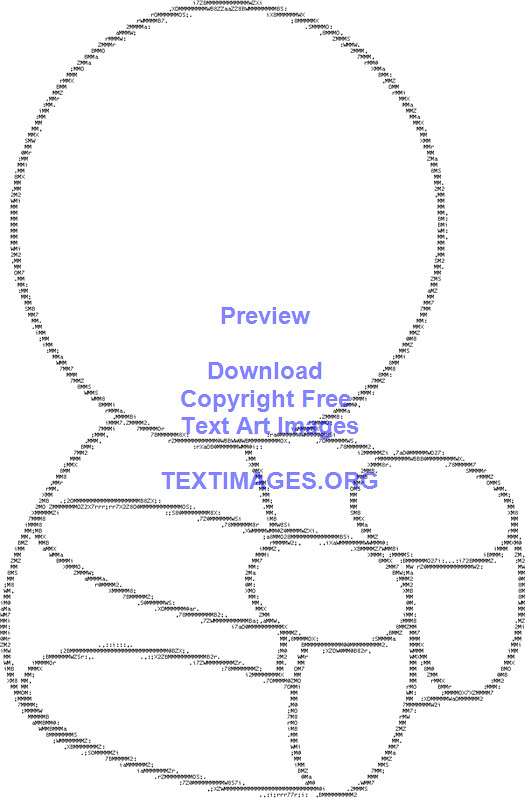In this image, a piece of text art depicts an extremely simplistic figure resembling either a stick figure or an outline of a teddy bear. The design consists of various basic geometric shapes: a round, empty circle represents the head, while the body is formed by an egg-shaped oval, and the limbs—arms, hands, legs, and feet—are all depicted with oval shapes. The figure appears to be in a seated position with its arms and hands extending towards its feet, which also rest in front. The entire figure is outlined in alternating blue and white lines. Centrally arranged blue text reads: "Preview," "Download," "Copyright Free," "Text or Images," and finally "textimages.org." The background is plain white, devoid of any other features.